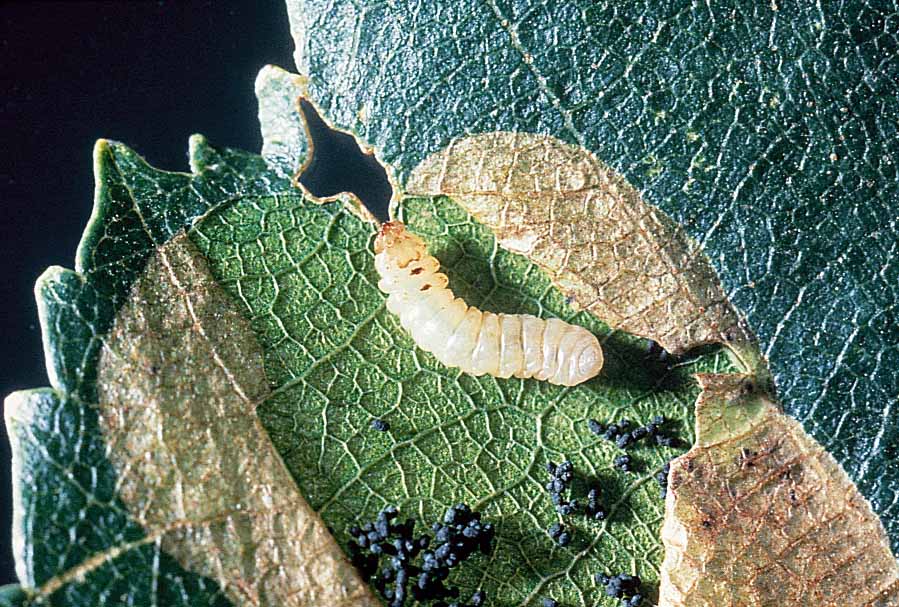The microscopic close-up image reveals an intricate view of a leaf set against a dark, almost black background. The leaf itself displays a spectrum of colors ranging from dark greenish-blue, brown, and tan to patches of bluish-green, and appears dry and weathered, exhibiting a cracked, leather-like texture. Prominently, the veins of the leaf are highly visible, adding to its intricate, veiny appearance. A small, white segmented worm or larva with a brownish-red head and two black spots is situated on the leaf, its body exhibiting a wrinkled texture. Surrounding the worm are approximately 30 to 40 black dots or small clumps that could be eggs or excrement. Additionally, eight holes perforate the leaf, contributing to its withered look, and there's a distinct glare from light reflecting off the leaf's surface.